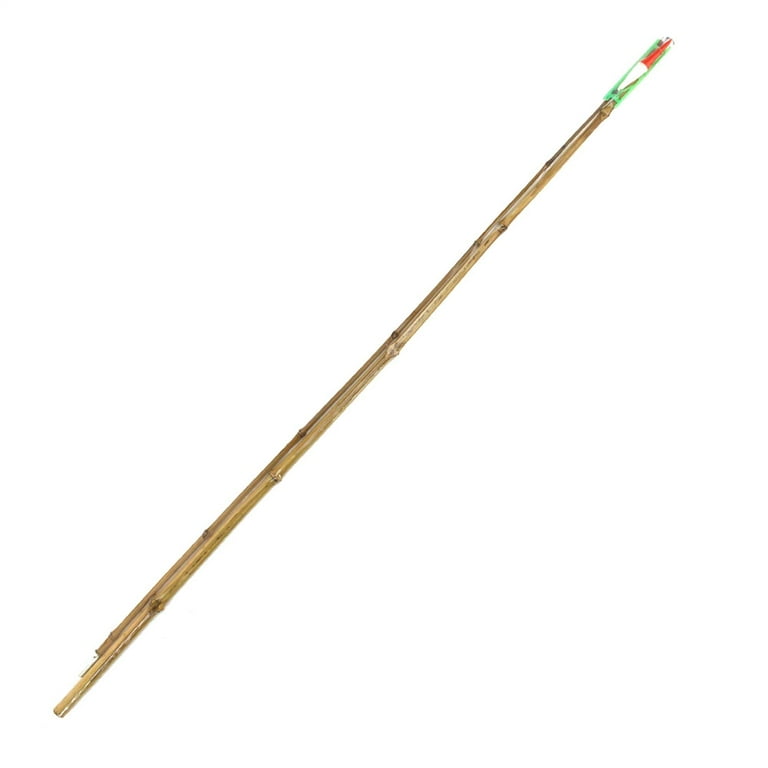The photograph features a long, thin wooden rod, resembling a dried piece of bamboo or possibly a branch, stretching diagonally from the bottom left to the top right of the image. The background is stark white, drawing attention solely to the rod. The wood appears blondish in color with a natural texture, displaying knots, tiny knobs, and dark brown circular features along its length, giving it an organic, uneven surface. One end of the rod is rough and seems slightly broken, while the other end is adorned with a bright green, transparent plastic piece. Nestled within this green piece is a long, diamond-shaped object with striking red and white sections, reminiscent of a fishing popper or possibly a component of a handcrafted tool. The intricate details suggest a combination of natural and synthetic elements, carefully arranged for an unknown, potentially utilitarian purpose.